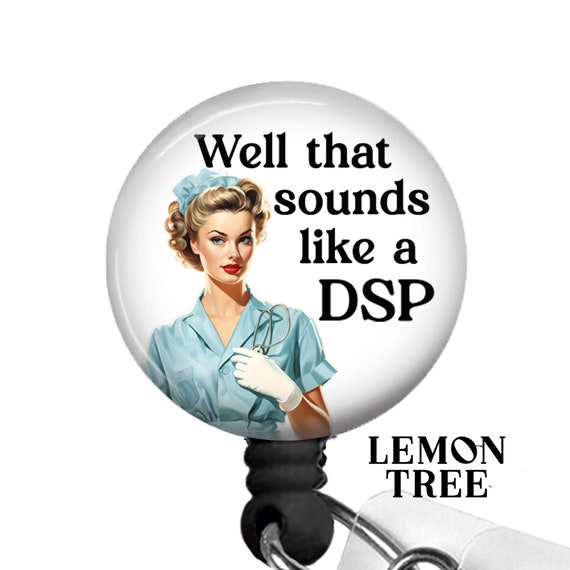This appears to be a circular pin or button on a white background, resembling an ornament, possibly meant for a lanyard. The pin features a vintage-style illustration of a woman with short, curly blonde hair tied up with a blue cloth or ribbon. She is depicted in a blue, short-sleeved nurse's outfit complete with white gloves and a stethoscope draped over her shoulder. The woman, who has applied full makeup including lipstick, is reminiscent of 1950s or 60s imagery. The top right corner of the circle contains the text "Well that sounds like a DSP" in black lettering. Below the circular part of the pin, there is a black base attached to a silver chain link, which connects to a piece of plastic, presumably part of a keychain. At the bottom of the pin, the words "LEMON TREE" are displayed in uppercase black text. This entire setup is positioned against a white background, suggesting that it might be an advertisement for a product.